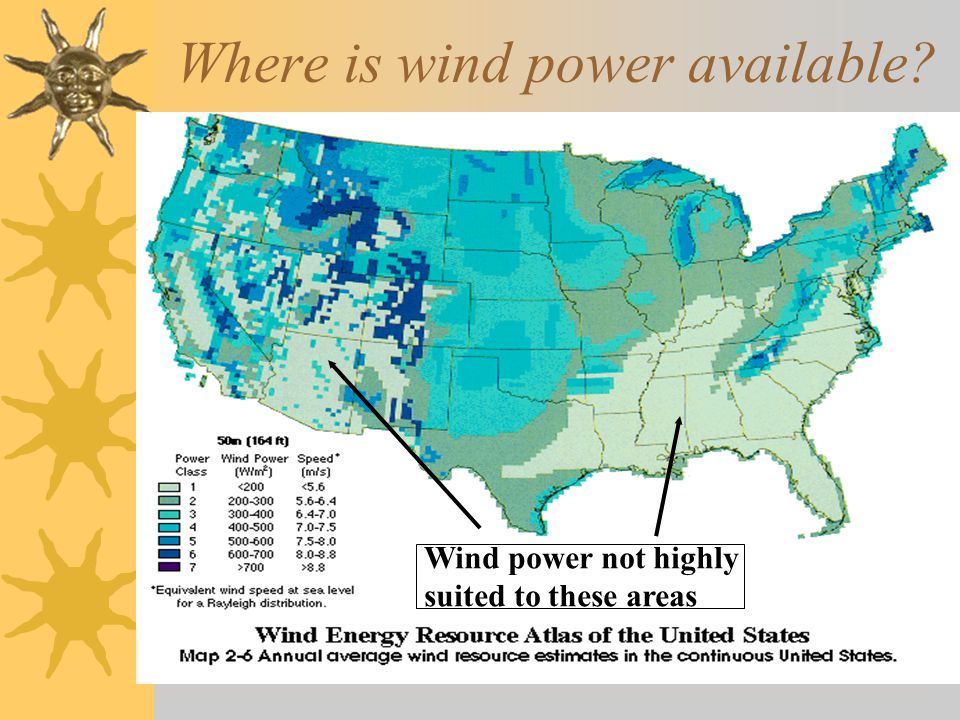The image is an educational infographic slide, primarily featuring a detailed map of the United States with state borders clearly outlined. The top of the map prominently displays the title in bold, brown letters: "Where is Wind Power Available?" The backdrop of the map is color-coded with various shades of blue, white, black, and gray to represent different wind power availability levels across the country. 

In the upper left corner of the map, the sun is visible, symbolizing energy. A significant portion of the dark blue shading, indicative of high wind power potential, is concentrated in regions just east of the Rocky Mountains. In contrast, the southeastern United States, including areas like Florida, features predominantly light shades like green and gray, indicating minimal suitability for wind power.

Beneath the map, text clarifies, "Wind power not highly suitable to these areas," with pointers directing to the least favorable regions. Additionally, there is a reference to the source of the map: "Wind Energy Resource Atlas of the United States, Map 2-6 Annual Average Wind Resource Estimates in the Contiguous United States." A chart or key on the map provides further explanation of the colors, with purple representing the highest wind power potential and light green denoting the lowest. This informative slide appears to be part of a PowerPoint presentation aimed at educating viewers on the spatial distribution of wind energy resources in the United States.